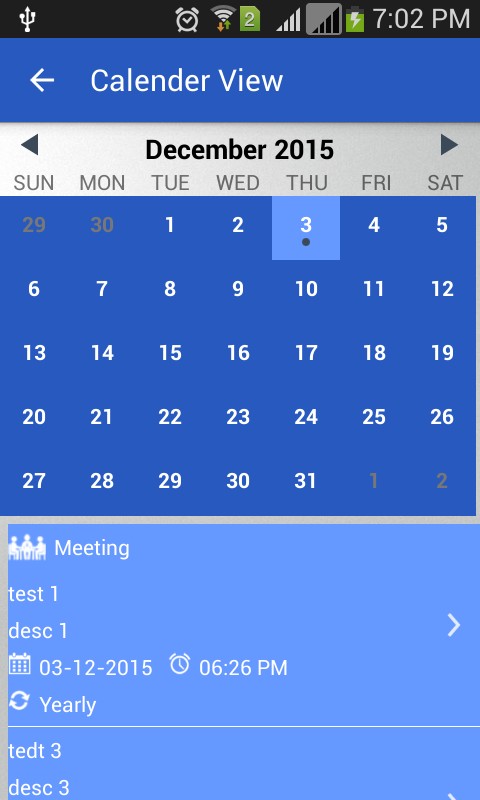This screenshot is from a mobile phone interface. At the very top, there's a black status bar featuring, on the left, a small white icon resembling connected wires. Moving right, there are icons representing an alarm clock, Wi-Fi signal, SD card status, and two mobile signal bars, followed by a battery icon with a thunderbolt symbol inside it. The time is displayed in white font as "7:02 p.m."

Directly below the status bar, there is a dark blue navigation bar with "Calendar View" written in white font in the center and a left-pointing arrow situated to its left. 

Beneath the dark blue bar is a white navigation bar with left and right arrows on either side. Centered between the arrows is "December 2015" written in black font.

Below this navigation bar, the days of the week (Sunday through Saturday) are displayed in gray font starting from the left to the right of the screen.

The main calendar grid follows, containing dates ranging from the 29th of the previous month to the 2nd of the following month, with the days numbered 1 through 31. The background of the calendar grid is the same dark blue as the navigation bar above.

Finally, at the bottom of the image, there is a lighter blue rectangle.